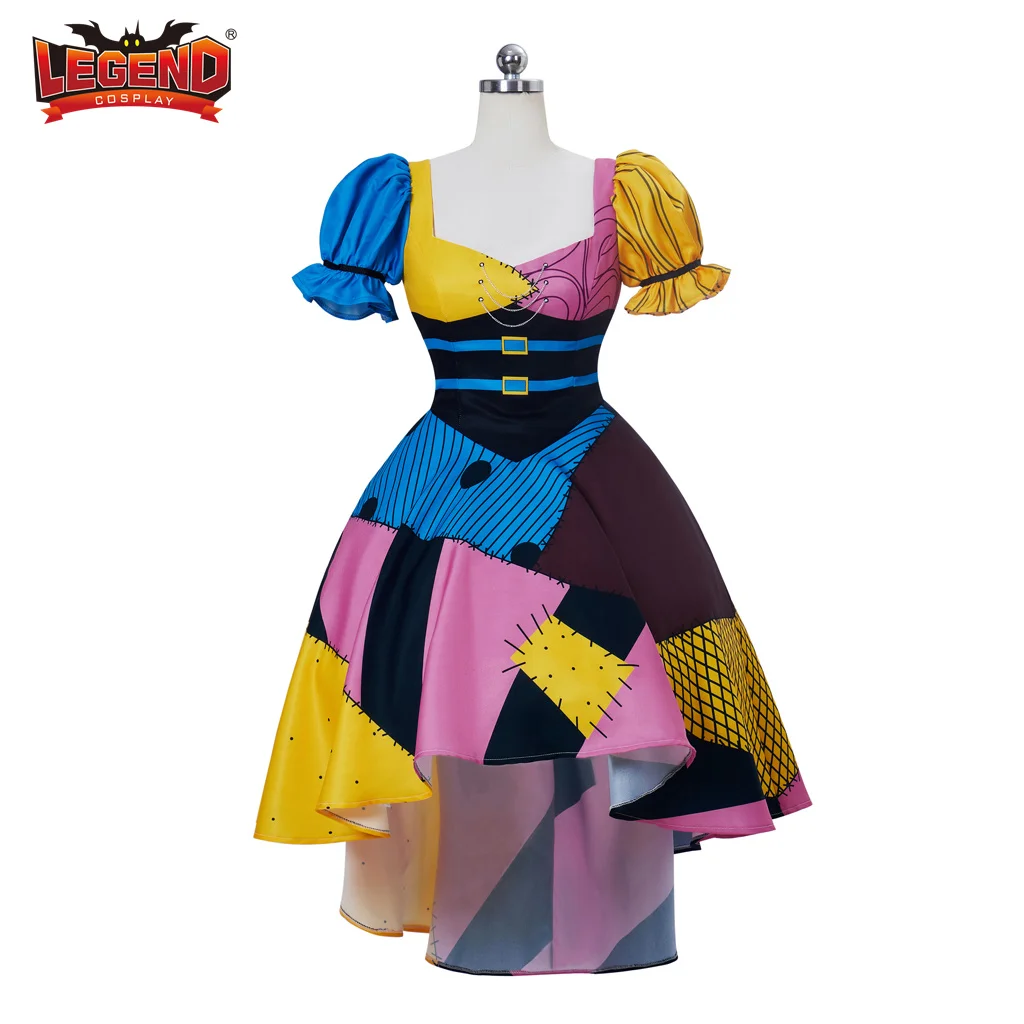The image displays a headless mannequin with a small metal bulb where the head would be, set against a solid white background. The mannequin is adorned in a vibrant and intricate costume, clearly inspired by a character from the movie "A Nightmare Before Christmas," most likely Sally. The costume features a patchwork dress displaying an array of different fabrics and patterns meticulously stitched together. The right sleeve of the dress is blue, and the left sleeve is yellow, both puffy and short-sleeved in a style reminiscent of a Snow White costume. The bodice showcases a mix of pink, yellow, black, and brown fabrics with two distinct blue belts across the waist. The skirt is an eclectic patchwork of colors including blue, brown, pink, black, and yellow, featuring a mix of stripes and polka dots. In the upper left-hand corner of the image, there is a logo of a black bat with yellow eyes, accompanied by the text "Legend Cosplay" in red lettering. The meticulous details of the outfit and the background suggest that this costume is designed for convincing character cosplay.